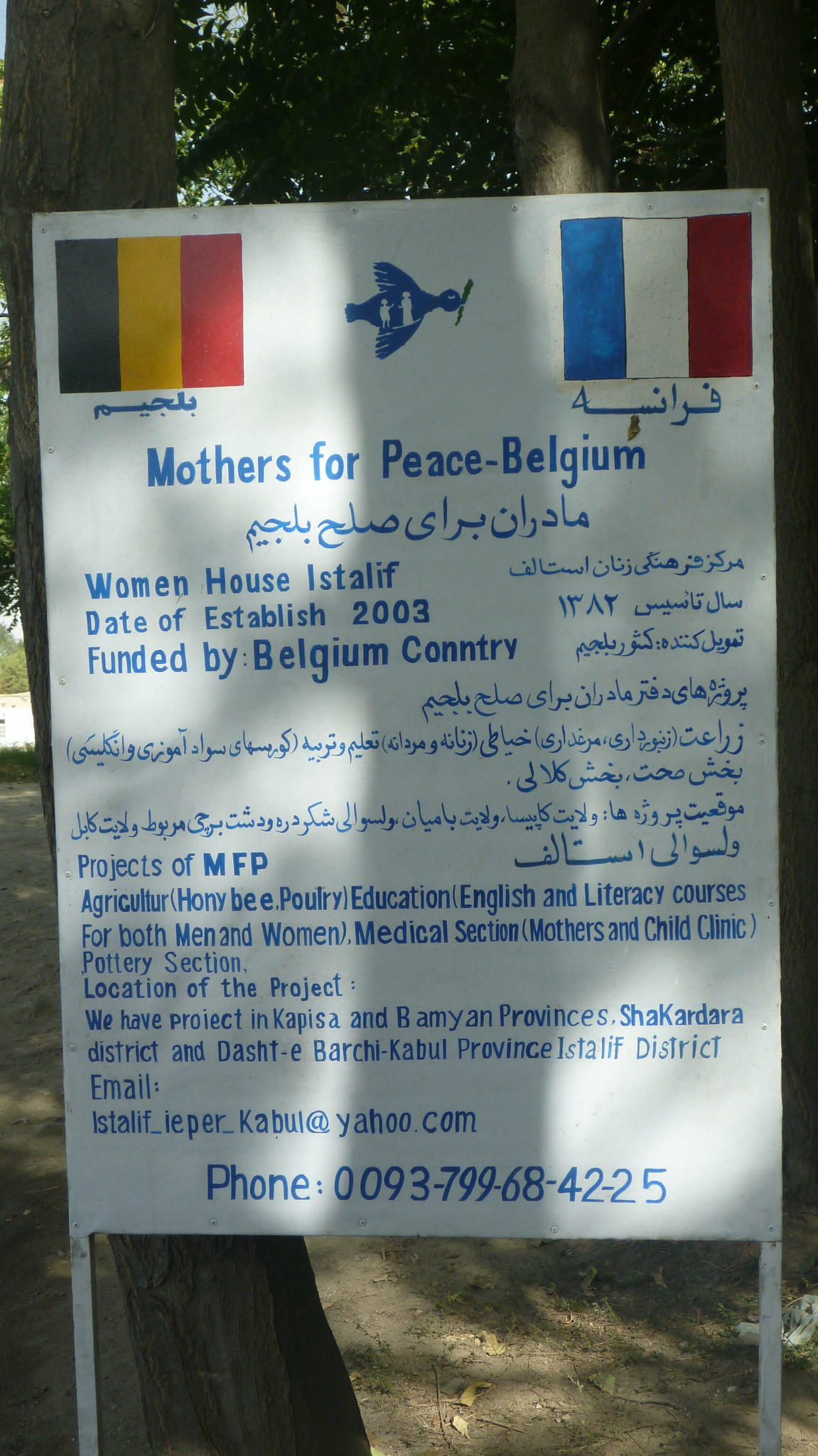The image depicts a large, white rectangular sign posted outdoors on two poles, situated in a wooded area. The sign features both English and Arabic text. At the top center of the sign, there's a blue illustration of a dove carrying a twig, which contains an image of two indistinct figures inside its outline. Flanking the dove are the Belgian flag on the left, with its vertical stripes of black, yellow, and red, and the French flag on the right, with its vertical stripes of blue, white, and red.

The sign’s header reads "Mothers for Peace Belgium" in blue letters. Below this, it states "Women House Istilove" and notes "Date of Establishment 2003, Funded by Belgium Country." The listed projects of Mothers for Peace include agriculture, honeybee cultivation, poultry, education, English and literacy courses for both men and women, a medical section, a mothers and child clinic, and a pottery section. The specific locations of these projects are identified as Capisa and Bamiyan Provinces, Shakadara District, and Dashti Barchi-Kabul Province in Afghanistan.

Additionally, the sign provides contact information, listing the email address as istilove-ieper-kabul@yahoo.com and the phone number as 0093-799-68-42-25. The entirety of the sign’s text is rendered in blue, making it visually consistent and easy to read against the white background.